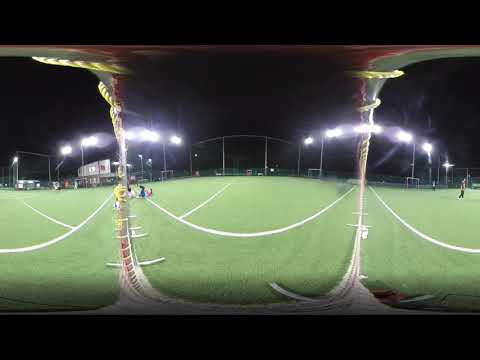The photograph captures a nighttime scene on a distorted soccer field, taken with a lens that alters the spatial characteristics of the terrain. The field appears empty, apart from a few people scattered in the distance, with some on the left side behind a bar-like structure in the foreground. This bar, wrapped with string or thread, stands out close to the lens. On the far right of the image, an individual stands alone near the edge.

The primary visual feature is an illusion created by the lens - what looks like ropes or lines stretching from both sides of the photo, forming a large U-shape that curves down and up through the field of vision. The field is illuminated by two rows of lights on the left and right, leaving the background in darkness. Despite its seeming simplicity, the image becomes an intriguing abstraction due to the distortive effect of the lens, giving it an almost surreal quality.